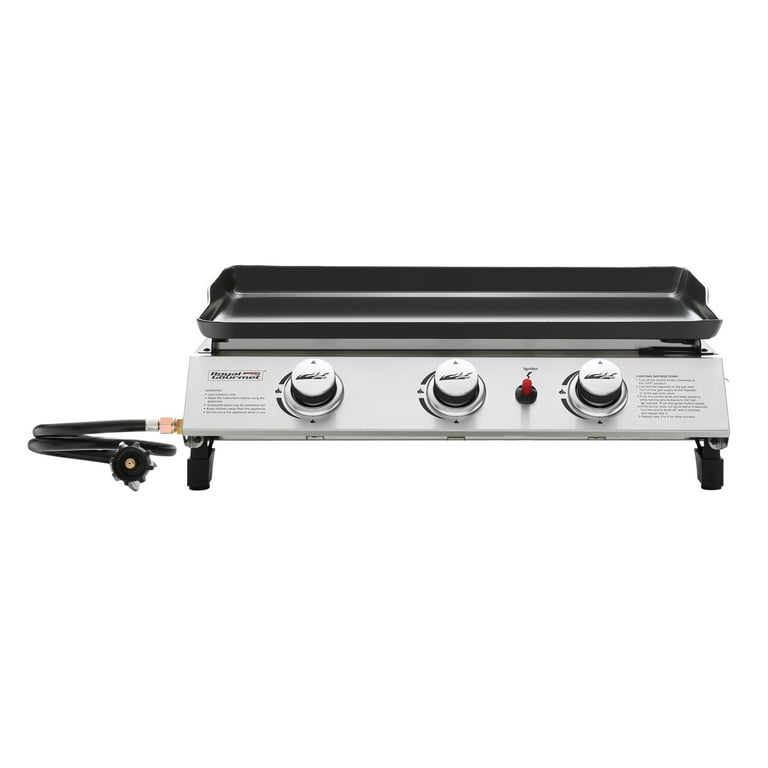This image portrays a portable cooktop featuring a sleek silver body and a flat black grill on top, ideal for cooking items such as hamburgers or pancakes. The cooktop is equipped with three metallic knobs, each adorned with black rubber rings, positioned on its front for easy manipulation. Notably, between the two rightmost knobs is a small red lever, which functions as an igniter button. On the left side of the cooktop, a black tube extends outward, featuring a brass fitting designed for connecting to a propane tank. The cooktop stands on four sturdy metal feet, each fitted with black rubber stoppers to prevent slipping. This device, which likely bears the brand name “Gourmet,” is situated against a white background.